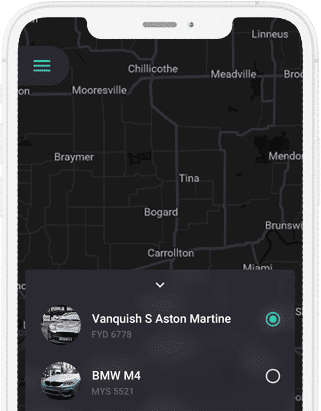Here is a cleaned-up and detailed caption based on the provided description:

---

Screenshot of the rideshare app prototype during testing, likely formatted for an iPhone interface. The main screen features a map displaying the user's current location and intended destination. Below the map, there are selectable car options, each with a corresponding image and probable license plate information. The first option is an Aston Martin Vanquish S, and the second is a BMW M4. Users can choose between these cars for their ride. Additionally, a menu button appears on the side, although it is a closed tab with no visible options in this screenshot.